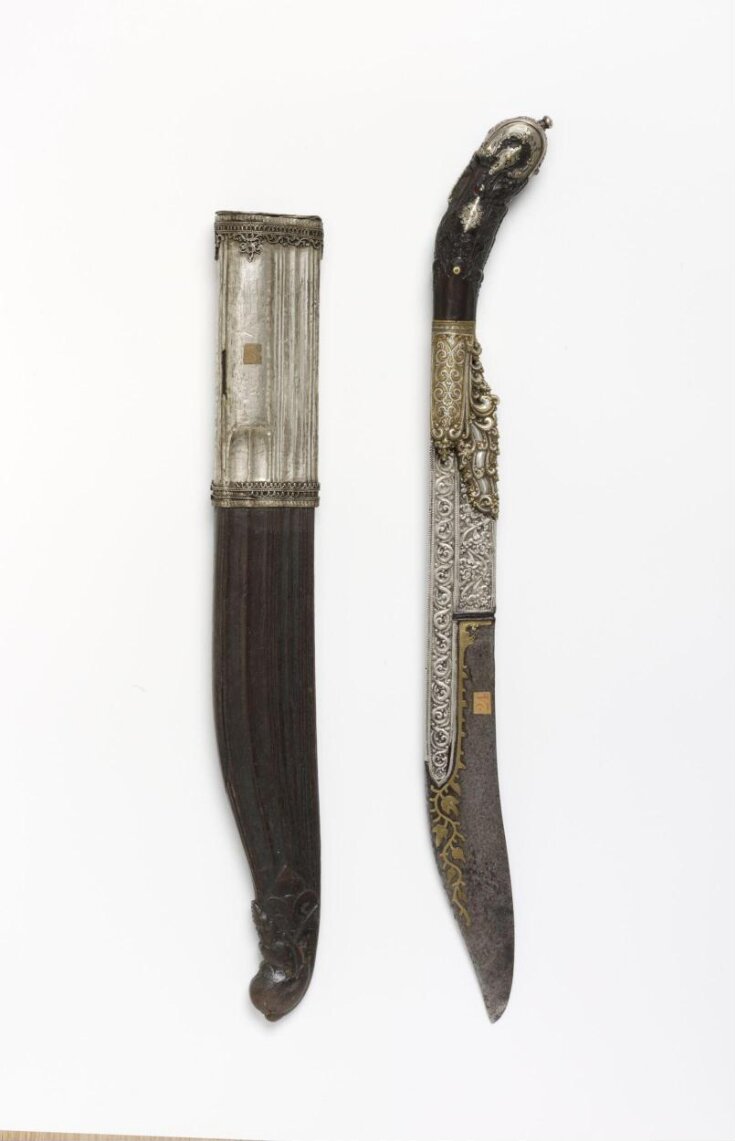This image depicts a photograph of an antique and ornately carved dagger along with its sheath. The backdrop is a plain white surface, which emphasizes the intricate details of the objects. The dagger, positioned on the right side, features a curvaceous, short silver blade adorned with elaborate carvings at the top. A striking gold leaf pattern enhances the upper section of the blade, seamlessly blending into a handle that combines different materials and decorations. The handle begins with a silver section showcasing a scroll design, followed by a gold band that replicates the same pattern, and culminates in a dark black leather grip. The handle is capped with a silver piece at its end. On the left, the sheath mirrors the dagger's ornate style. It features a silver top and a black leather body, meticulously crafted to match the dagger's aesthetic. Both pieces lie parallel to each other, highlighting the dagger's historical and artistic significance.